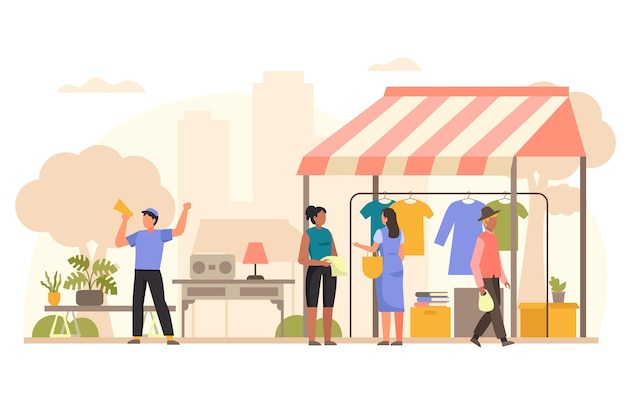The illustration vividly portrays a bustling outdoor shopping scene set against a backdrop of skyscrapers and trees, giving the ambiance of a vibrant city marketplace. Central to the image are two women engrossed in conversation, surrounded by an array of colorful clothing. The woman on the left is dressed in a blue and black outfit, clutching a white top, while the woman on the right wears a blue dress and carries a yellow purse. A clothes rack next to them brims with hanging garments in shades of blue, yellow, and green, neatly sheltered under a pink and white canvas canopy resembling a small tent.

To the right side of the canvas, a man in a pink shirt, adorned with a lighter pink long-sleeved layer underneath, and black trousers, strides by, donning a black cowboy-style hat. Meanwhile, positioned on the left side of the illustration is another man, animatedly promoting goods. Dressed in a blue short-sleeved shirt, black trousers, and a blue hat, he holds what appears to be a megaphone to his mouth, gesturing energetically with a yellow object in his hand. In front of him, a table displays various home appliances, including a boombox and a lamp with a pink shade. Adding a touch of nature, a potted monstera plant sits at the leftmost edge of the scene.

This detailed depiction captures the essence of urban shopping, with people engaged in lively exchanges amid a diverse mix of products and greenery, all under the expanse of a dynamic cityscape.